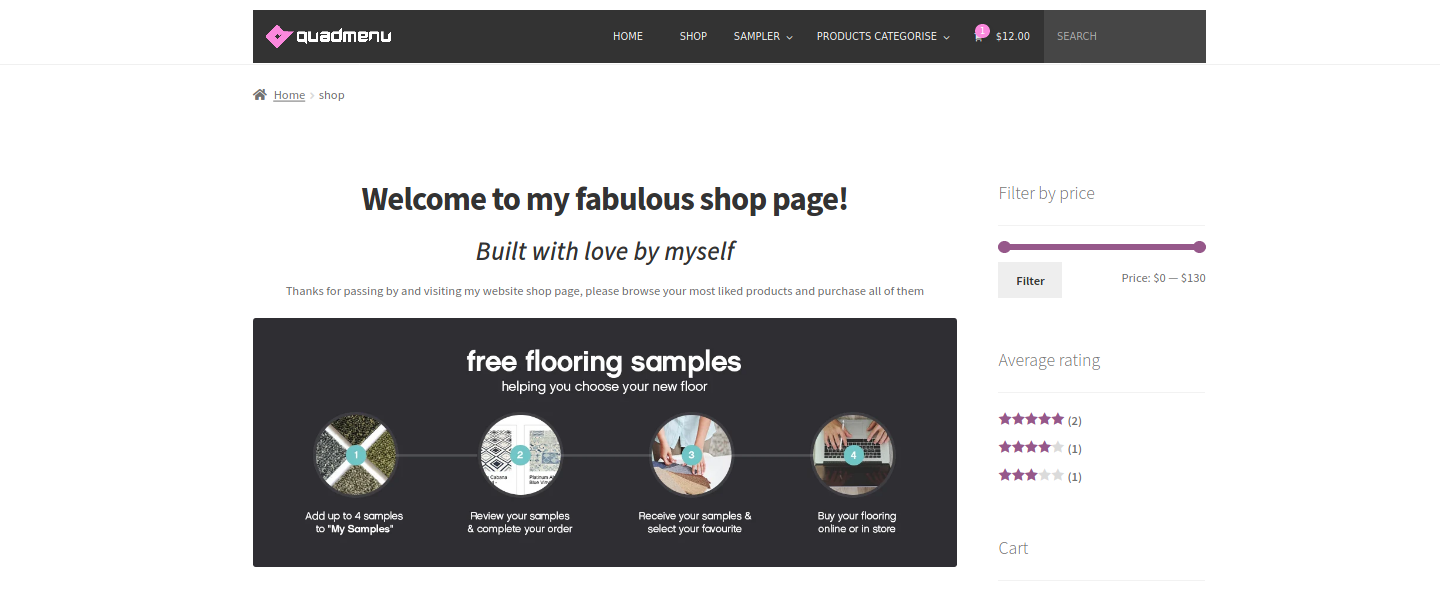At the top of the interface, a prominent header labeled "Quad Menu" is displayed, featuring a design resembling a purple ticket. The menu includes various options such as "Home," "Shop," "Sampler," "Products," and "Categories." Below it, a circular button, also in purple, is labeled "$12." 

In a contrasting green hue, a search bar is provided with the label "Search." Further down, text on the page welcomes visitors with the message, "Welcome to my fabulous shop page, built all by myself." This is followed by a note of appreciation: "Thanks for passing by and visiting my website shop page. Please browse your most liked products and personalize your look."

On the top right corner, a section dedicated to filtering by price is highlighted, with purple accents. Adjacent to this, a gray filter button allows users to refine their product search by various price points ($7 or $2.30) and their average ratings (5 stars, 2 items; 4 stars, 1 item; 3 stars, 1 item).

A large gray rectangle dominates the center of the display, containing text that reads, "Free Florid samples, helping you choose your new Florid." Instructions are provided to add items to the Florid homepage and manage samples: "All that's left is to add up to Florid's homepage, to my samples, then X." Additional guidance advises, "Review your samples and complete your order," and encourages, "Save your samples and select your favorite. Here are our top four."

Concluding the display, a call to action invites visitors to "Buy your Florid online or in-store."